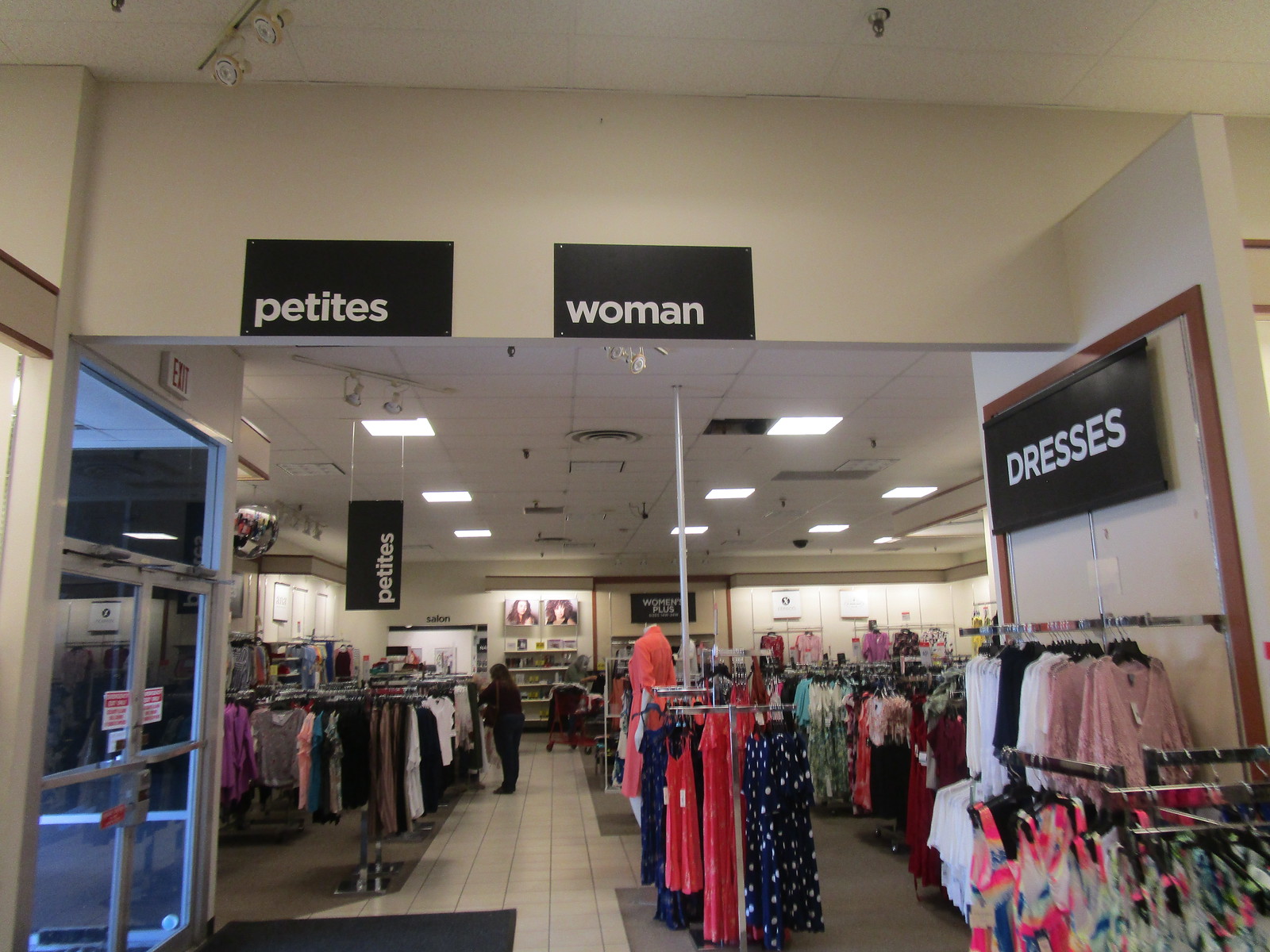This image depicts the interior of a women's clothing store with a minimalist aesthetic marked by plain white walls and a combination of white tile and low-pile industrial carpet flooring. The store is illuminated by square beams of light on a tiled ceiling, casting spotlights that somewhat bleach out the finer details of various signs and images.

Several prominent black signs with white lettering categorize different sections of the store, including "Petites," "Women," and "Dresses." In the rear of the store, there's also a section labeled "Women Plus." These signs contribute to an organized shopping environment, although specific brand logos and stock images of models are present but difficult to read due to the strong lighting.

The store features a variety of clothing racks displaying an array of garments in numerous colors, including pinks, purples, whites, blues, and dark shades, as well as items with polka-dot and flowery prints, suggesting no single seasonal theme. Sparse decorations and a practical layout dominate the setting.

Two emergency exit doors, labeled with a red "EXIT" sign and cautionary warnings, are located on the left side of the image, indicating a strict adherence to safety protocols.

Amidst the merchandise, a shopper browses through the aisles, and further back, a store clerk can be observed, enhancing the image of a bustling retail environment.